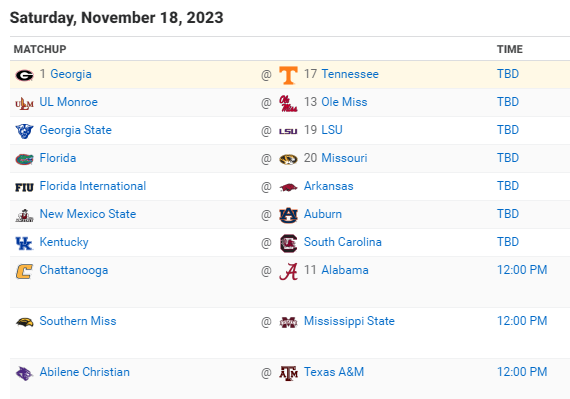**Detailed Basketball Game Schedule for Saturday, November 18, 2023**

The image displays a neatly organized schedule for basketball games on Saturday, November 18, 2023. The schedule is presented in three columns, each distinctly marked with bold black headings. 

**Column Headers:**
1. **Match-Up:** The first column lists the symbols representing different basketball teams.
2. **Teams:** The second column displays the corresponding opposing teams.
3. **Time:** The third column indicates the scheduled time for each game, highlighted in capital blue letters.

**Details:**
1. **Match-Up:** Georgia vs. Tennessee
   - **Time:** TBD
2. **Match-Up:** UL Monroe vs. Ole Miss
   - **Time:** TBD
3. **Match-Up:** Georgia State vs. LSU
   - **Time:** TBD
4. **Match-Up:** Florida vs. Missouri
   - **Time:** TBD
5. **Match-Up:** Florida International vs. Arkansas
   - **Time:** TBD
6. **Match-Up:** New Mexico State vs. Auburn
   - **Time:** TBD
7. **Match-Up:** Kentucky vs. South Carolina
   - **Time:** TBD
8. **Match-Up:** Chattanooga vs. Alabama
   - **Time:** 12 PM
9. **Match-Up:** Southern Miss vs. Mississippi State
   - **Time:** 12 PM
10. **Match-Up:** Abilene Christian vs. Texas A&M
    - **Time:** 12 PM

This schedule keeps fans informed of their favorite team match-ups and the timing of each game, ensuring they won’t miss any action on this jam-packed day of basketball.